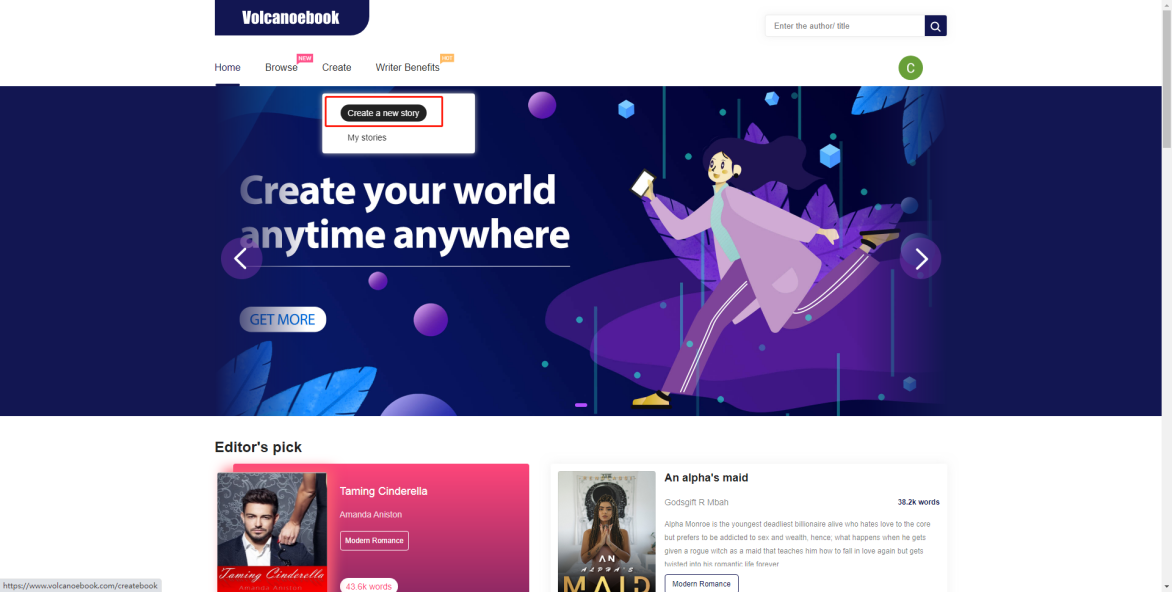The image depicts the homepage of a book website named "Volcano Book," prominently displayed in white text on a dark blue background at the top left. Below the website name, there are four categories listed horizontally: Home, Browse, Create, and Writer Benefits. The "Browse" category is highlighted with a pink rectangle featuring a white logo, while the "Writer Benefits" category is also highlighted, but with a yellow rectangle.

At the top right corner of the page, there is a search bar with placeholder text that reads "Enter the search title." Directly beneath the search bar, a green circle with a white letter "C" is visible.

The central portion of the image features a cartoon illustration of a woman running to the left. She is depicted wearing purple pants, yellow shoes, a pink jacket, and a green shirt. To the left of the cartoon woman, the text reads, "Create your world anytime, anywhere." Furthermore, at the bottom left corner of this central section, there is a caption that says, "Get more."

At the very bottom of the overall image, two book covers or products are displayed. The product on the left showcases an image of a man and is titled "Taming Cinderella." The product on the right is titled "The Alpha's Maid."